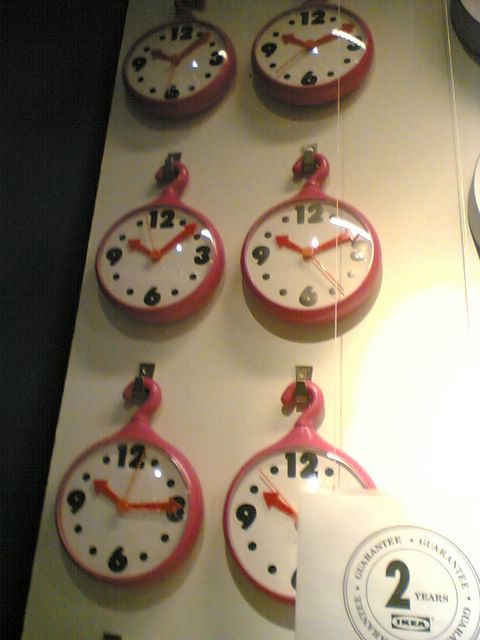The image features a white background, resembling a wall, with a section of black adjacent to it. Prominently displayed on the white wall are six red clocks, each featuring a hook at the top for easy hanging. The clocks are uniform in design, with red clock hands and minimalist faces that highlight only the numbers 12, 3, 6, and 9, using dots to mark the remaining hours. A sticker at the bottom of each clock reads "IKEA guaranteed 2 years." The clocks display different times: one shows approximately 10:05, another around 10:10, a third indicates between 10:20 and 10:25 (partially obscured by a sticker), one is set to 10:15, and another is nearly at 10:15.